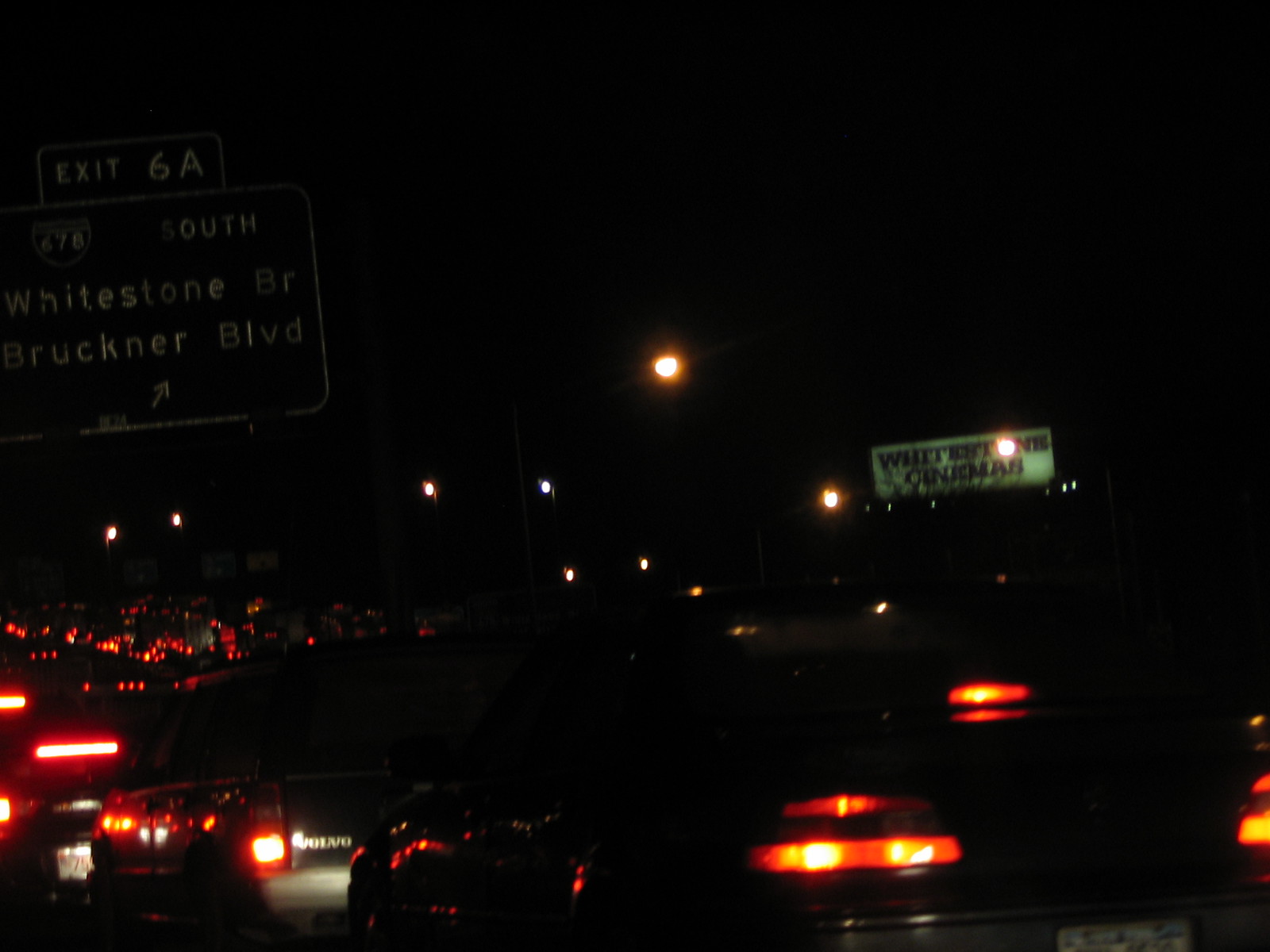The image captures a bustling nighttime scene outdoors, marked by a myriad of car lights concentrated on the left side towards the background. Dominating the top left corner, two signs are visible; the smaller upper sign clearly reads "EXIT 6A," while the larger, partially obscured lower sign displays directions that include "SOUTH," "Whitestone," "BR," and "Bruckner Boulevard," with an upward-pointing arrow. To the right in the background, a billboard stands silhouetted against the night sky, adding to the urban atmosphere of the scene.